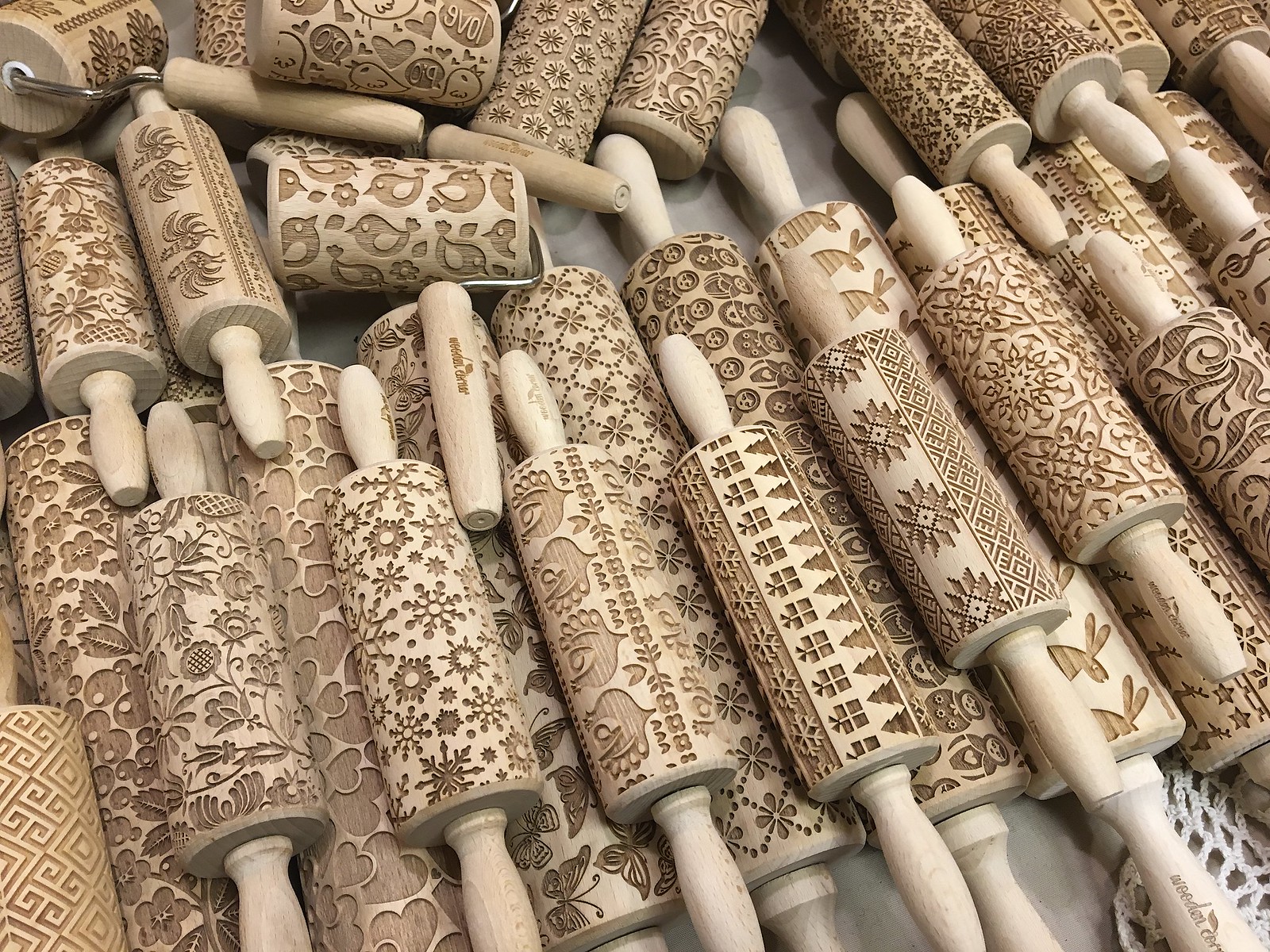In this image, a plethora of intricately designed wooden rolling pins are scattered across a gray surface. There are at least 25 to 30 rolling pins, each featuring unique and busy patterns meticulously carved into the wood. The designs vary from Christmas-themed motifs, such as presents and snowflakes, to more nature-inspired elements like birds, bees, flowers, trees, leaves, and even chickens. 

The rolling pins exhibit a wood-like brown color with darker hues accentuating the carved patterns. Some rolling pins include words like "love" and heart shapes. Additionally, a few handles are equipped with silver metal or wire details, adding a touch of craftsmanship.

The layout of the image shows larger rolling pins at the bottom, stacked horizontally in rows, with smaller ones placed on top, extending diagonally across the image. The top left corner of the photo features another prominently placed rolling pin. The designs are repeated across the collection, making the scene appear very busy and visually engaging.